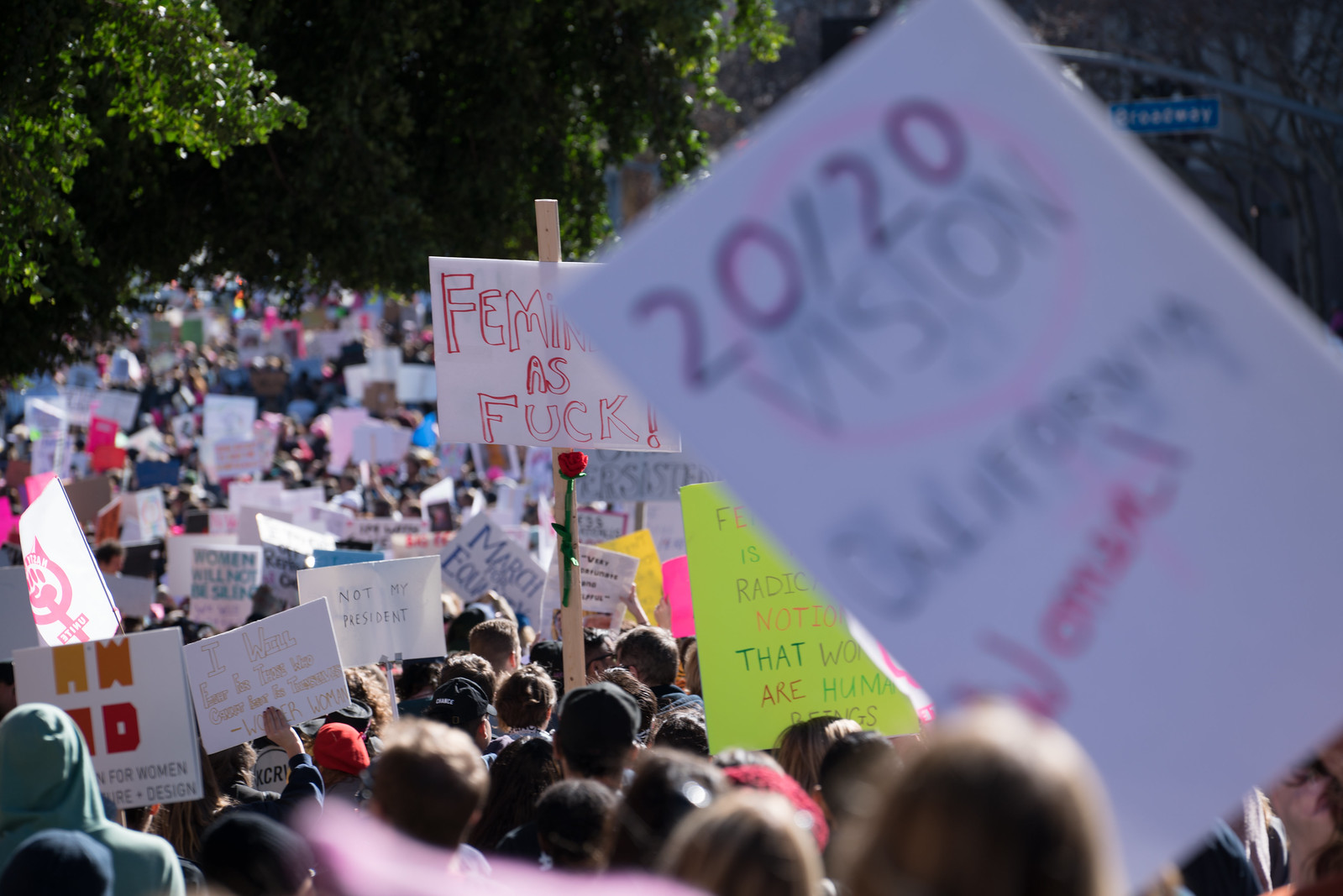This image captures a large outdoor daylight protest, stretching into the distance with a diverse crowd filling the frame. Predominantly focused on women's rights, many of the participants hold signs, adding a vibrant and colorful element to the scene. One prominent sign in the foreground reads "2020 Vision," albeit slightly out of focus, and another nearby boldly states "Feminist as Fuck." A bright green sign further declares "Women are Human Beings," reinforcing the rally's theme. The protestors, seen from behind, include varied attire such as hats and hoodies, all marching down a tree-lined street. Dense greenery and branches from a tree hang over from the left, creating a scenic backdrop. On the right, an out-of-focus blue street sign and a streetlamp are barely discernible. Among the multitude of signs, messages advocating for gender equality and political statements like "Not My President" add to the intensity of the demonstration. Despite the multitude of signs, many remain unreadable in the image, leaving a rich mosaic of activism and solidarity on display under the open sky.